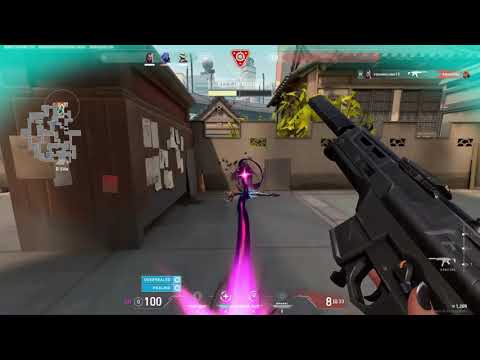The image is a screenshot from a first-person shooter video game, featuring a scene with the player's character holding a black automatic rifle in their right hand. The character appears to be female, indicated by the black nail polish on their fingernails. A striking magenta or pink beam or laser extends from the character, shooting directly forward, while a faint lime green hue, possibly from leaves, appears in the background. The scene is set in an outdoor area with various structures. To the left is a wooden-paneled wall adorned with scattered papers, while a brown building with a green-tinted roof or aura looms in the far distance. On the right side of the image, there is a concrete or stone fence behind which some leaves are noticeable, suggesting nearby foliage. The top and bottom of the image are bordered by black bars, and a white map with various directional icons is visible on the far left. Other game HUD elements are present, including a health indicator displaying '100' with a plus symbol at the bottom. A turquoise green light also appears in the top part of the image, adding to the intricate visual details of the game environment.